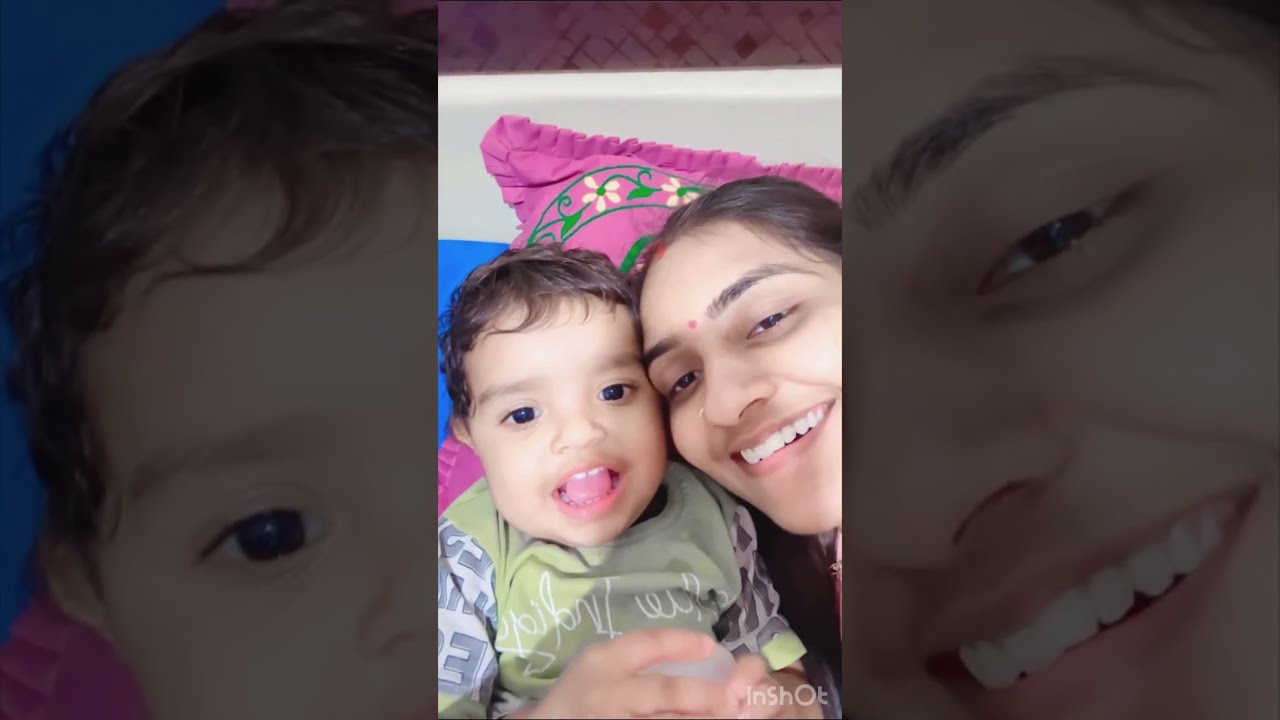In this image, a young Indian woman and a baby are closely huddled together, both staring directly into the camera with joyful expressions. The woman is on the right, featuring a prominent pink dot between her eyebrows on her forehead. She has brown eyes, brown eyebrows, and brown hair. Her mouth is open in a wide, bright smile, showcasing her upper row of teeth. Beside her, the baby mirrors her joyful expression, with its mouth open wide, revealing upper teeth, a tongue, and pink lips. The baby also has brown eyes and short, slightly fringed dark hair. Behind them is a pink pillow embellished with green stems and white flower bulbs. The baby is dressed in a light green shirt with white lettering and gray "E"-shaped patterns on the sleeves. The bottom right corner has the word "In Shot" visible in shadow, indicating the photo-editing app used. The image is flanked by two zoomed-in sections; the right side focuses on the woman's eye and part of her mouth, while the left side highlights the baby's left brown eye. The background appears to be a bed with additional pillows, accentuating the cozy and intimate setting.